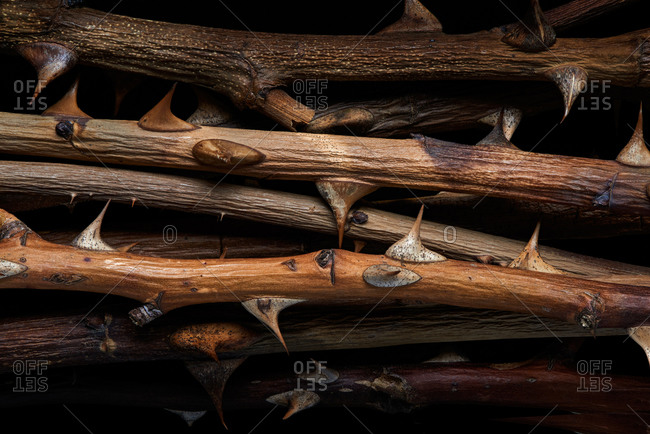This image features an array of thin, thorny branches laid out in a parallel fashion against a background covered in shadow. At the very top, there's a dark brown branch with tiny white specks along its surface, slightly obscured by shadows. Prominently displayed thorns jut out from the left side of this branch. The words "O-F-F" and "1-3-5" appear in light gray near the thorns and at various other points across the image, creating a diamond-shaped pattern overlay.

Beneath this, a slightly lighter brown branch with a burn mark on the right side has thorns mostly on the left. Below, a medium brown branch showcases numerous small thorns scattered along its length. Moving down further, you'll notice another branch of lighter brown wooden color, adorned with large gray thorns that extend from top to bottom.

Towards the middle of the arrangement, a smaller lighter brown stick with tiny thorns can be observed, followed by a chestnut brown, shiny branch boasting prominent thorns. Near the bottom, two additional branches are visible, the lowest possessing a reddish hue and also bearing thorns.

Overall, the branches exhibit a diverse palette of brown tones—ranging from light tan to dark brown, some even appearing burnt. The entire composition is accentuated with varying sizes of sharp, pointy thorns, creating an intriguing textured contrast against the shadowy backdrop.